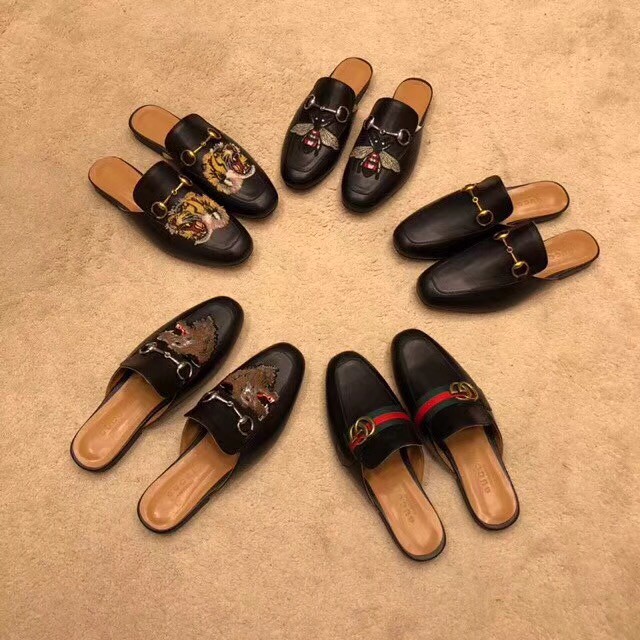In this indoor photo taken on a beige carpet under artificial lamp lighting, we see an arrangement of five pairs of black backless loafers formed in a circle. Each pair features a distinct decorative design on the top. One pair is plain with a traditional gold buckle. Another pair showcases a striking design with a gold beetle adorned with a red body and wings extending outward. A third pair depicts a fierce lion with its mouth open, accompanied by gold hardware. The fourth pair has a gold wasp or cicada emblem, and the final pair is embellished with a green and red stripe resembling a Gucci print, completed with two gold circles. All pairs share the characteristic tan soles, giving them a unified appearance despite their unique decorations.